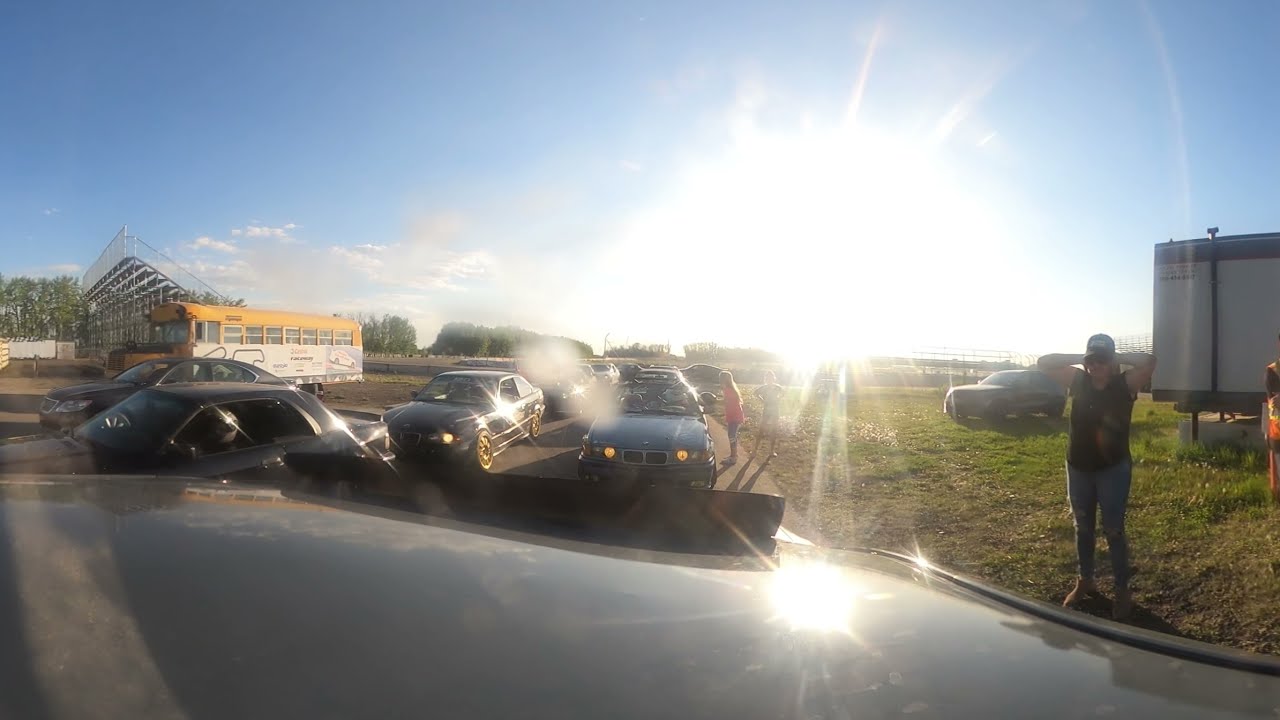A photograph captures a sunny scene at the edge of a parking lot or field, possibly near a high school stadium, given the visible bleachers and a yellow school bus angled on the left. The image is taken from inside a vehicle, as indicated by the slight blur at the bottom of the windshield. In the foreground, sunlight creates a distortion on the shiny exterior of a car, altering its usual shape. At the right-hand side stands a person, possibly a man, wearing blue jeans, a black short-sleeved shirt, and a baseball cap. This individual has their arms behind their head and is near a grassy area. Behind them, a car is parked and there is a trailer toward the middle-right of the image. The scene is bustling with multiple cars, some lined up in two lanes of traffic, while others are parked around. The bright white sun casts a significant glare across the picture, illuminating the green grass and a clear blue sky, further enhancing the bright and lively atmosphere.